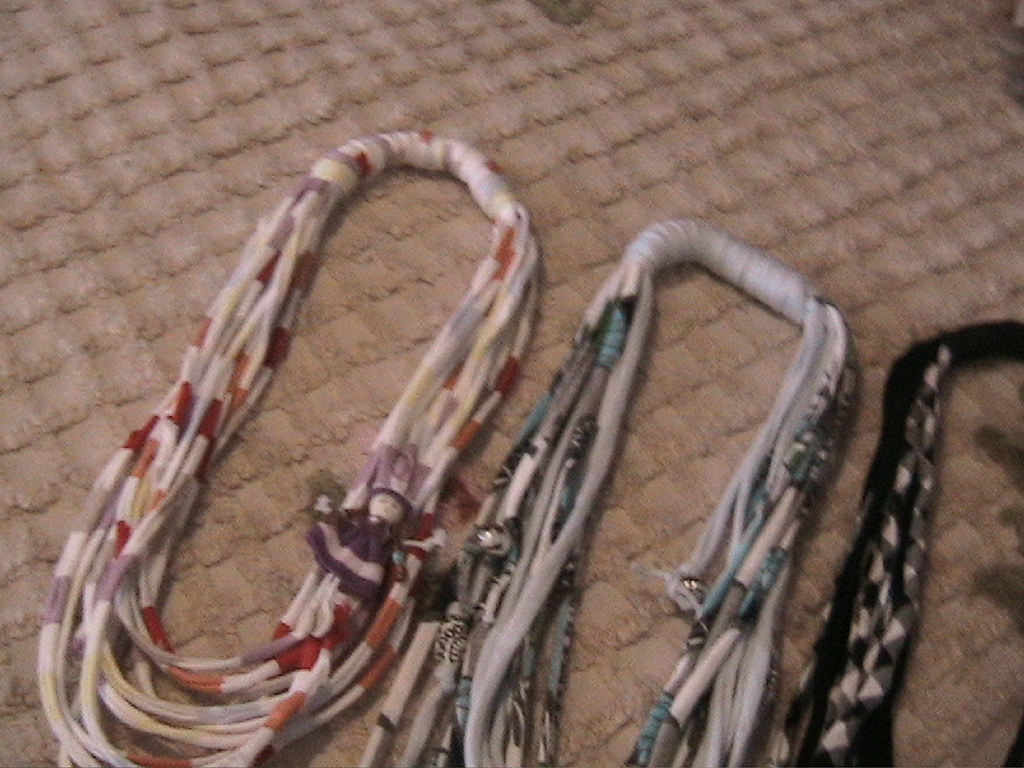This detailed photograph showcases three intricately designed necklaces set against a light beige carpet with a raised square pattern. The necklaces exhibit tribal or indigenous artistry, featuring multicolored strings with alternating bands of color. The first necklace, positioned on the left, consists of strings in a white, orange, white, red, and white sequence, tightly woven into a long, thin oval shape. This piece also includes a small purple doll affixed to it. The middle necklace alternates between teal and white stripes, ornamented with silver beads or bells, adding to its intricate design. The rightmost necklace, only partially visible, displays a black base with beige triangle patterns. Each necklace merges many strings into a single cohesive piece, demonstrating both unity and complexity in their construction.